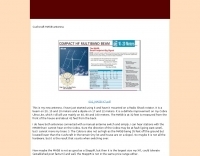The image appears to be a document or webpage layout that is quite blurry, making the specific text unreadable. The background is divided into three sections: light peach on the left and right sides, and a white central area. At the very top and center of the image, there is a dark burgundy bar that does not extend to the edges of the page. Below this, the main content area begins.

On the upper left corner of the white section, there is some black text. Positioned centrally below this area is a box containing an image accompanied by a caption or title in black text above it. Adjacent to the box with the image, there is a blue bordered box that features white text.

Further down, there is a sketch or illustration that appears to be primarily blue and white, with additional text located to its right. Directly beneath this section, there is a chart composed of formatted text with light blue content and a dark blue header. To the right of this chart, a gray bordered box encloses some additional text.

At the bottom of the image, more black text is laid out in paragraph format, consisting of at least three distinct paragraphs. Each section appears to be a continuation or perhaps part of a larger document, though the exact details due to the blurriness remain indiscernible.